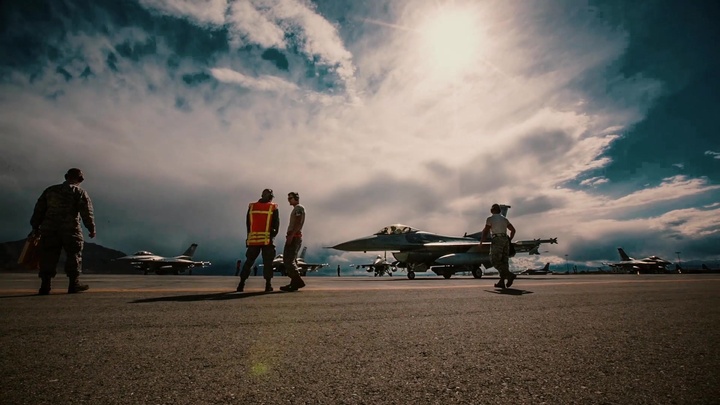The image depicts a scene on a military air force base runway featuring four men in the foreground. The man on the far left dons a gray army uniform, reminiscent of soldier attire, while the second man, standing to his right, is outfitted in a bright orange vest with yellow lines and a hard hat. To the right of him, a man in a red shirt appears engaged in conversation with another man, who is farthest to the right, wearing gray work pants and a white t-shirt, running towards a nearby jet. The background reveals six silver military jets, with one front-most jet preparing for takeoff, a pilot visible in the cockpit. The runway is gravelly, and the sky above is blue with significant cloud cover, the sun shining through, casting a bright yet somewhat shadowy atmosphere.